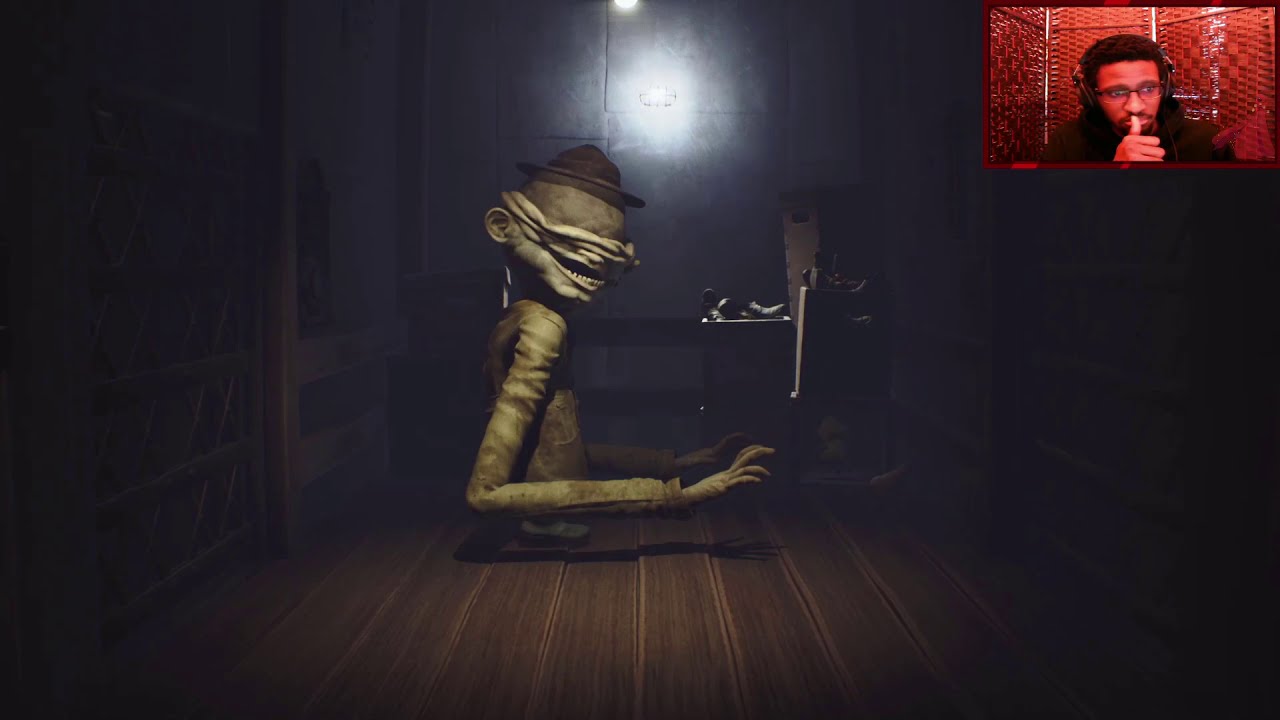The image is a still from a video game depicting a dark and eerie room with wooden floors, largely enshrouded in shadows. Light from a single source near the ceiling casts a spotlight on a peculiar creature sitting in the center. The creature has an unsettling appearance with a grayish-brown body consisting of a torso with feet, but no legs, and exceptionally long, skinny arms. It wears a funny little hat on its bald head and a blindfold over its eyes, revealing a wide, toothy mouth with far too many teeth. The dim light highlights the creature's face and part of the floor, while the rest of the image fades into darkness, adding to the creepy ambiance.

In the upper right-hand corner of the image, a small inset shows the gamer, who appears to be another vlogger. The gamer's room is bathed in a reddish light, making everything appear tinted red. He has black hair, a beard, glasses, and a mustache, and is wearing a black sweater. He is thinking deeply, with his thumb up near his nose, while sitting in a room with noise-canceling foam panels in the background. The gamer's hand is raised as if expressing an idea or reaction to the game. The eerie visual and the reddish tint of the gamer's webcam feed contribute to the unique and unsettling vibe of the overall image.